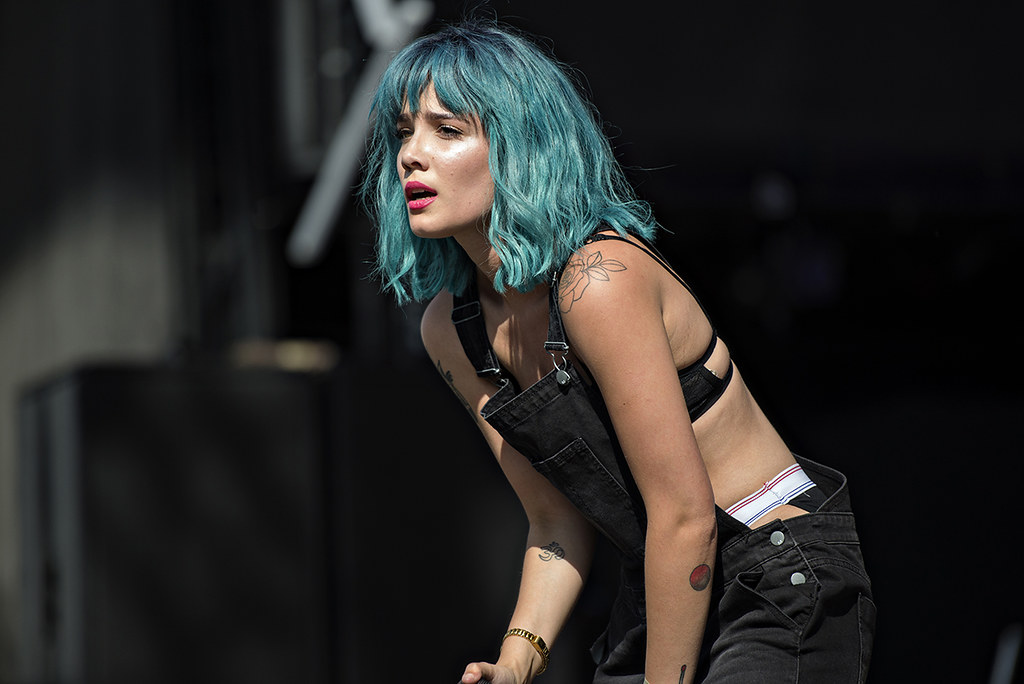In this image, a young woman, possibly in her mid-twenties, with striking turquoise hair, leans forward slightly, her left hand touching her inner thigh. Her hair frames her face, which displays an intense expression with slightly closed eyes and an open mouth, as if she's singing or speaking. She is clad in black overalls with shoulder straps fastened by buttons in the front, and a visible black bra underneath. She wears a gold bracelet on her bent right arm and a regular watch on her left wrist. Her outfit reveals a white-banded pair of underwear rising above the waistline of her overalls. Her lips are coated in bright red lipstick. The background is blurred and dark, creating a stage-like atmosphere with indistinct shapes that could be large speakers, hinting she might be performing. Her tattoos, including four on her arms, add to her distinctive appearance.